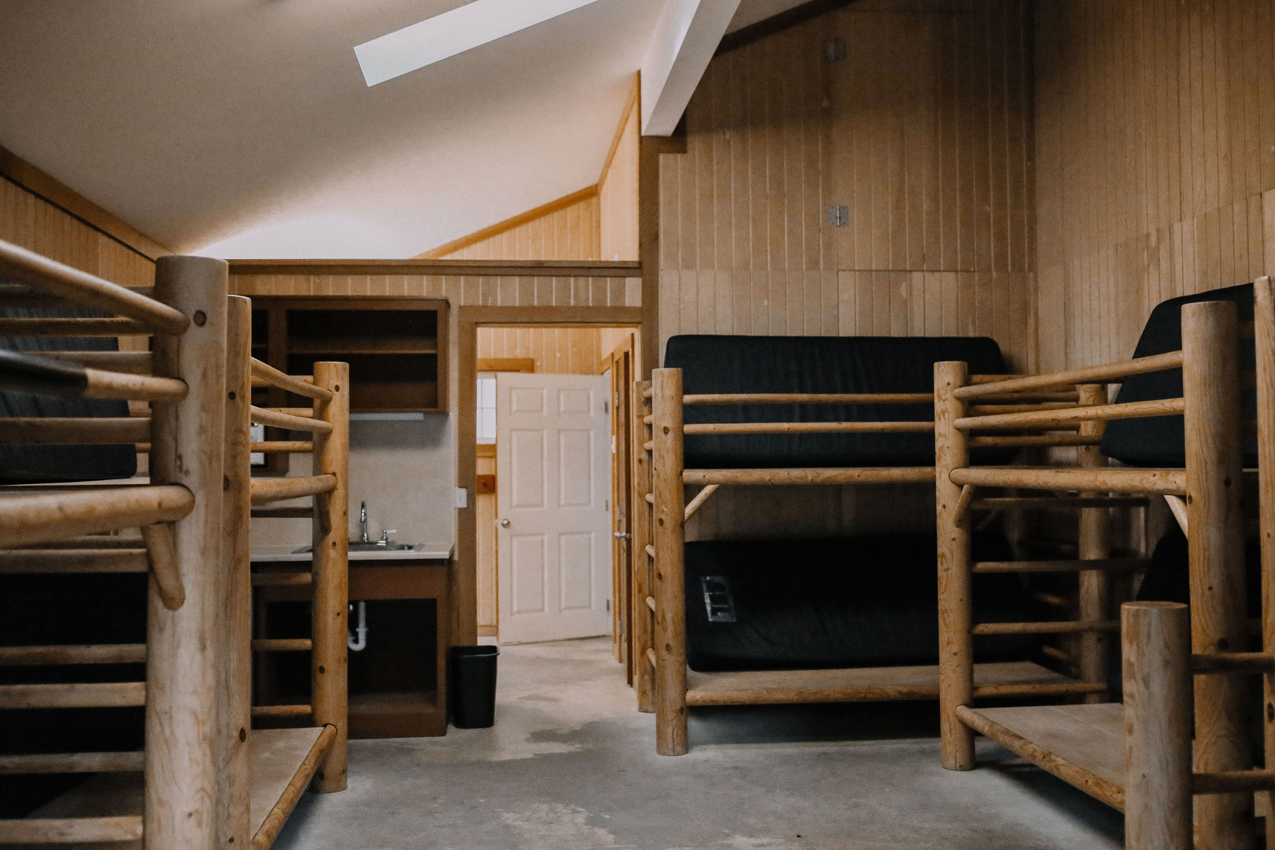A rustic, cabin-like room is depicted, with wooden bunk beds and walls that exude a warm, natural charm. The ceiling contrasts in white but is also accented with wooden beams. The room contains four sets of bunk beds in total, with two sets along the right wall and two sets on the left, one slightly cut off in the image frame. In front of the left-side bunk beds, there is a white countertop with a brown wooden surface. It features a silver faucet with white handles, and the white pipe beneath it is visible, adding to the room's functional yet cozy atmosphere.